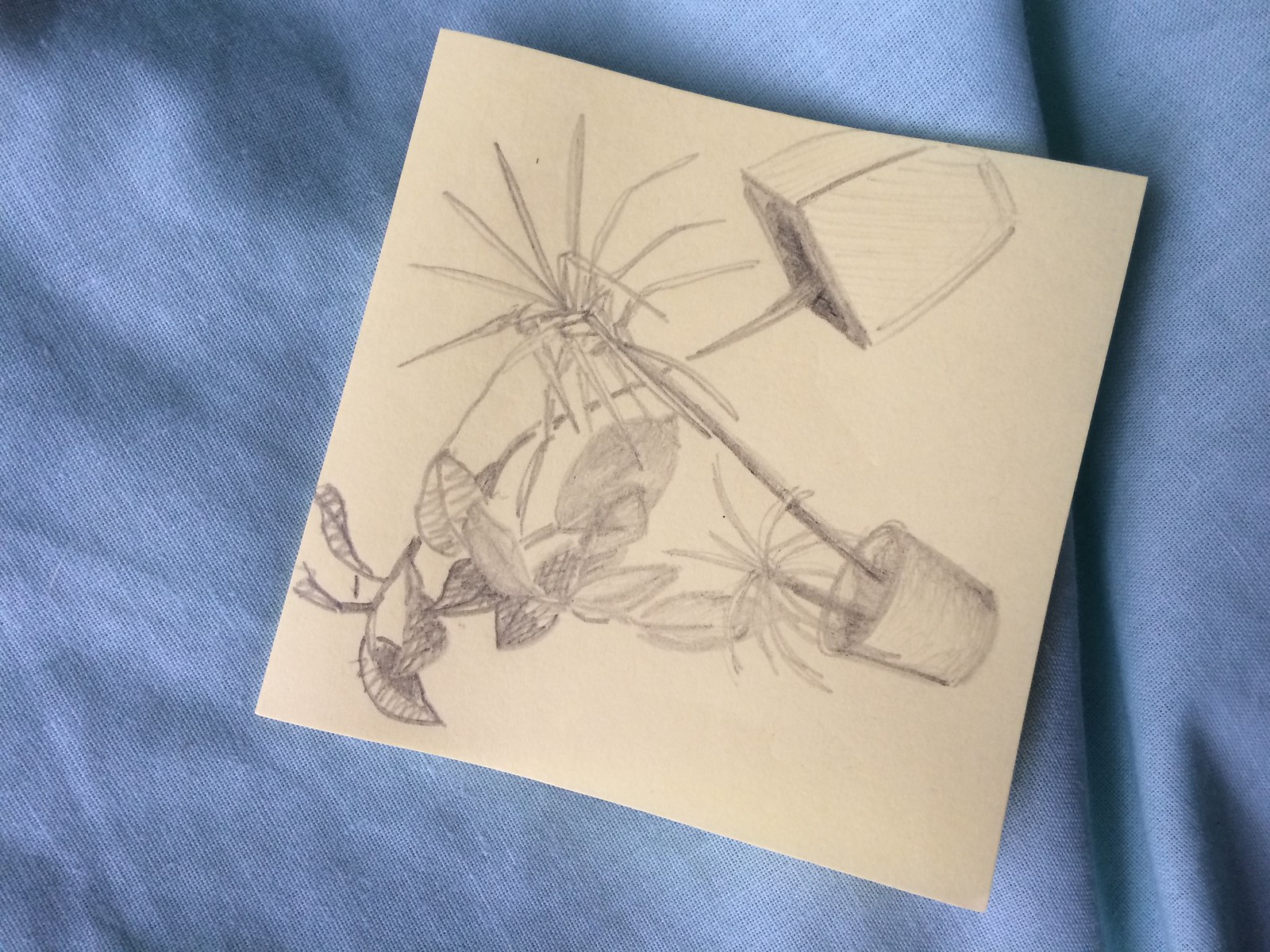This is a photograph of a detailed line drawing on a square piece of beige or tan paper, placed at an angle on a blue cloth background. The drawing is done in grayscale, using either sketch pencils or charcoal, and it depicts two potted indoor houseplants. One plant, originating from the right side of the paper, features oval-shaped leaves, while the other plant, which appears to be more tropical and palm-like, has thin, elongated fronds and intersects perpendicularly with the first plant. The drawing exhibits good solid shading, making the plants' forms and textures evident. Despite the rough, sketchy appearance, the artist's skill is apparent in the clarity and detail of the plants. The paper and plants are slightly overlapping in the composition, adding depth to the image.